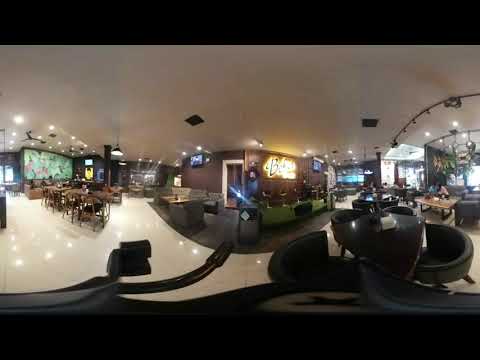The image depicts the interior of a lobby area, which appears to double as a bar or restaurant. The foreground features black circular seats arranged on a white, glossy tile floor. The overall image is somewhat distorted, particularly at the top and middle sections, giving a rounded and warped appearance. Moving to the right, there's a couch for seating near a table with a beige marble top, with more black circular chairs positioned to the left.

To the right edge of the frame, a large glass partition can be seen with plants hanging in front. In the middle of the scene, there is a counter resembling a bar or front desk area, and above it, a sign with glowing yellow letters, though the specific text is blurry, only the letter "B" is discernible. Towards the left side, another seating area is visible, including a wall-mounted TV and additional brown tables with matching chairs. The space is enclosed with white walls and a ceiling, while the side walls are brown, adding to the warmth of the interior.

Color details include a mix of black, tan, yellow, green, white, orange, and brown tones, contributing to the inviting atmosphere of the restaurant-like setting. The scene is captured as if during the middle of the day with ample indoor lighting. Despite the image's distortion, it's clear that this is a bustling, multi-functional space designed for comfort and social interaction.